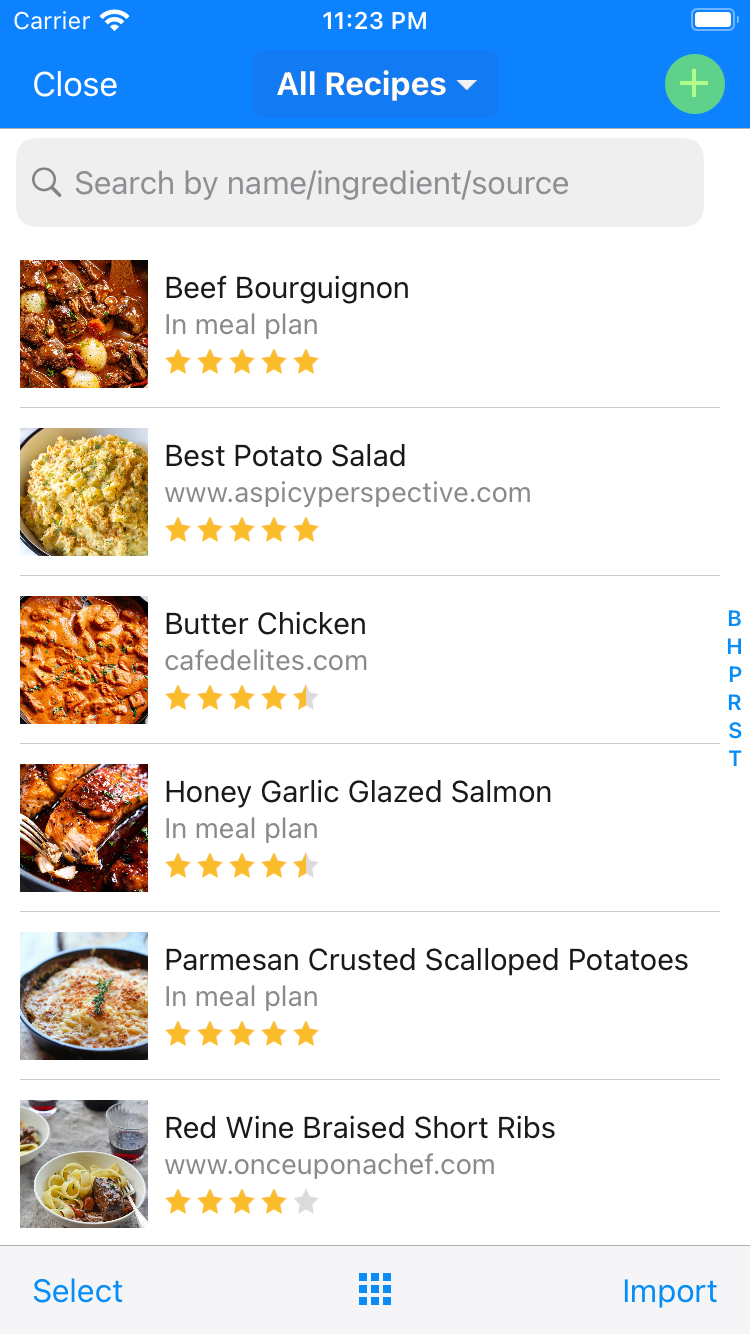The image showcases a screen capture from a mobile phone displaying a recipe collection interface. At the top of the screen, a drop-down menu currently set to "All Recipes" is visible. Below this, a search bar allows users to search recipes by name, ingredient, or source. The main portion of the screen lists several recipes, each accompanied by an image on the left side, the recipe title, a link to the full recipe, and the star rating given by users. The recipes displayed in order are:

1. Beef Bourguignon
2. Best Potato Salad
3. Butter Chicken
4. Honey Garlic Glazed Salmon
5. Parmesan Crusted Scalloped Potatoes
6. Red Wine Braised Short Ribs

Each recipe entry features a corresponding image on the left and an alphabetical index on the very right, indicating an option to sort the recipes alphabetically. At the bottom of the screen, there is a secondary menu with three options: an item selector on the left, a grid-style view button in the center, and an "Import" text button on the far right.